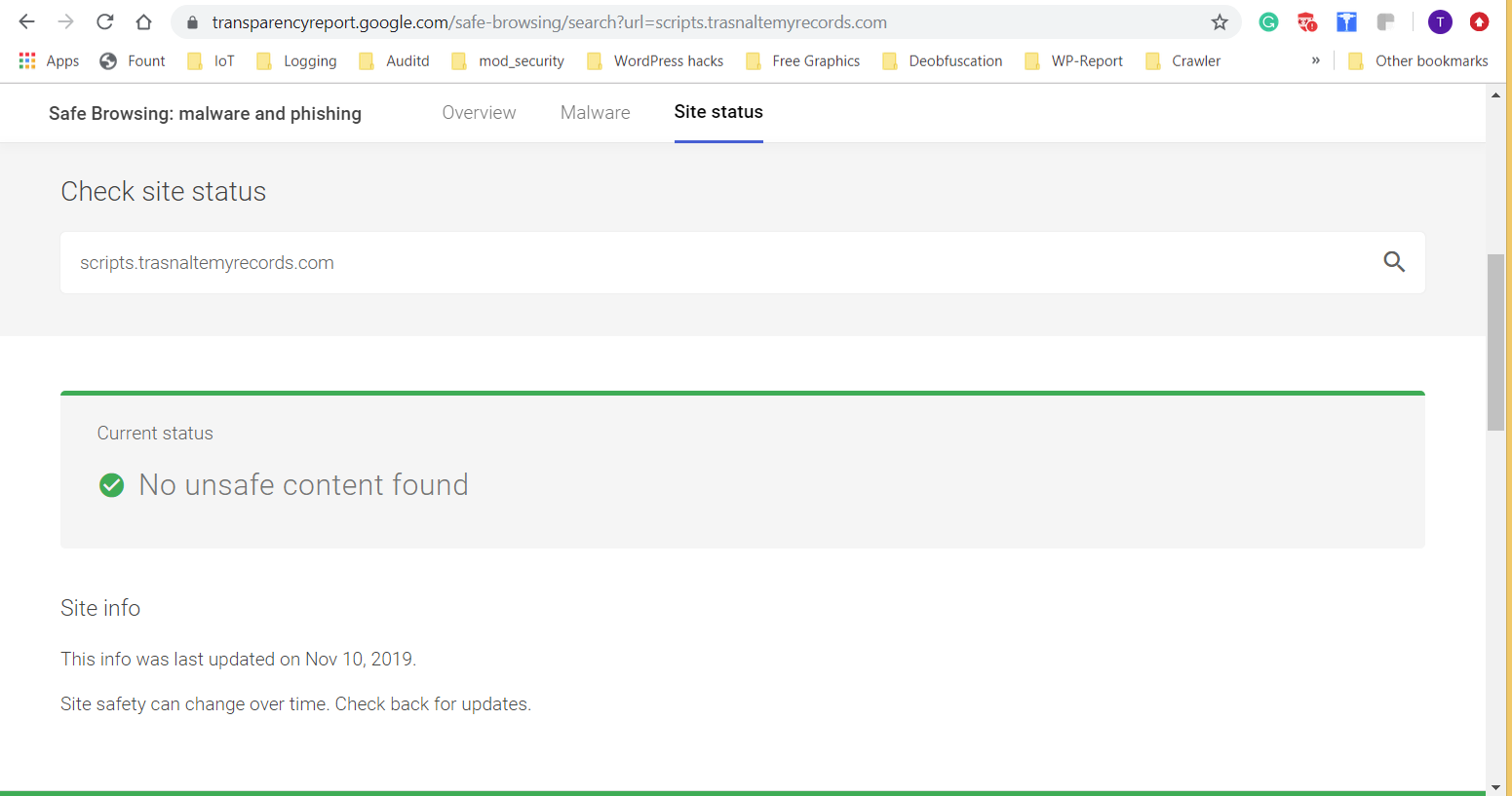**Detailed Caption:**

The image is a screenshot from the website "transparencyreport.google.com," specifically from the "Safe Browsing: Malware and Phishing" section. At the top, the navigation bar indicates several clickable sections, with "Overview," "Malware," and "Site Status" being prominently displayed. The "Site Status" tab is highlighted in black with a blue line beneath it, indicating it is the current selection.

Directly beneath the navigation bar, there is a gray rectangular box labeled "Check Site Status." Within this box, there is an input field containing the URL "scripts.transalteryrecords.com."

Below this, a green status bar is visible. Adjacent to it, the text reads "Current Status" next to a green circle containing a white check mark, indicating that no unsafe content was found on the site. Further down, a section titled "Site Info" provides additional details, noting that the information was last updated on November 10, 2019. A cautionary note follows, reminding users that site safety can change over time and advising them to check back for updates.

At the bottom of the image, a long, continuous green line further emphasizes the site's clean bill of health.